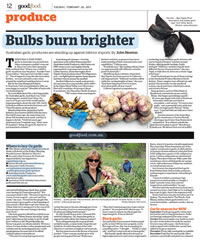Here is the cleaned-up and detailed caption:

---

The image showcases a small screenshot that appears to be from a digital magazine, characterized by a white background and challenging readability. The layout is reminiscent of an online magazine or newspaper article, segmented into distinct columns by thin gray lines. 

At the very top, there are various small and unreadable elements, starting with a "12" followed by the phrase "Good Food," among other text. Below this header, larger text spells out "Produce and Orange." Directly beneath this title, a dark banner line spans across the width of the image.

Subsequently, bold black text, highlighted as if manually, reads "Bold Burn Brighter." Under this prominent headline, the main article spans four columns, though the text is illegible. Central to the four columns, at their lower section, there is an image that seems to depict food.

Additionally, a picture of a woman standing in a farm field occupies the middle section of the layout. A horizontal black banner crosses the page further down, suggesting the continuation of the article beyond this point. The inclusion of images and structured columns of information hints at a comprehensive and visually engaging piece.

---